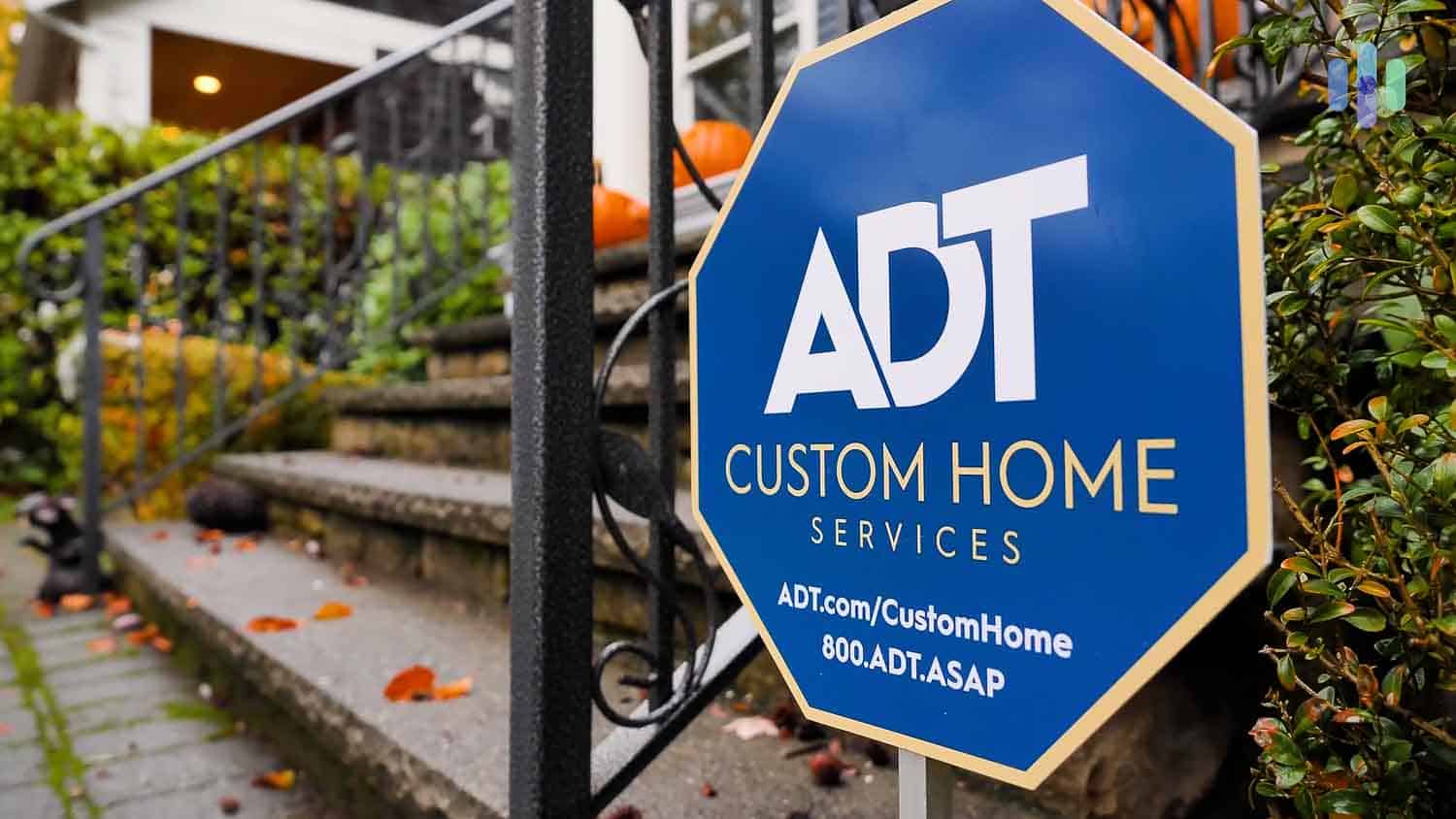The image captures a landscape-oriented view of a home security sign, prominently featuring the blue ADT Custom Home Services sign positioned near the steps of a house. The sign, octagonal in shape and reminiscent of a stop sign, has a medium blue background with a yellow trim. The large ADT logo in white letters is centrally placed, with "Custom Home Services" in smaller yellow letters below it. Further down, the URL "ADT.com/customhome" in white letters and the contact number "800.ADT.ASAP" are visible. The sign is situated in front of a lush green bush, which is to the right of a set of five or six cement steps leading up to a porch. These steps have black railings on each side. Additionally, there's a brick walkway with moss growing between the bricks in the foreground of the house. In the background, other elements of the house and neighboring buildings can be faintly seen.